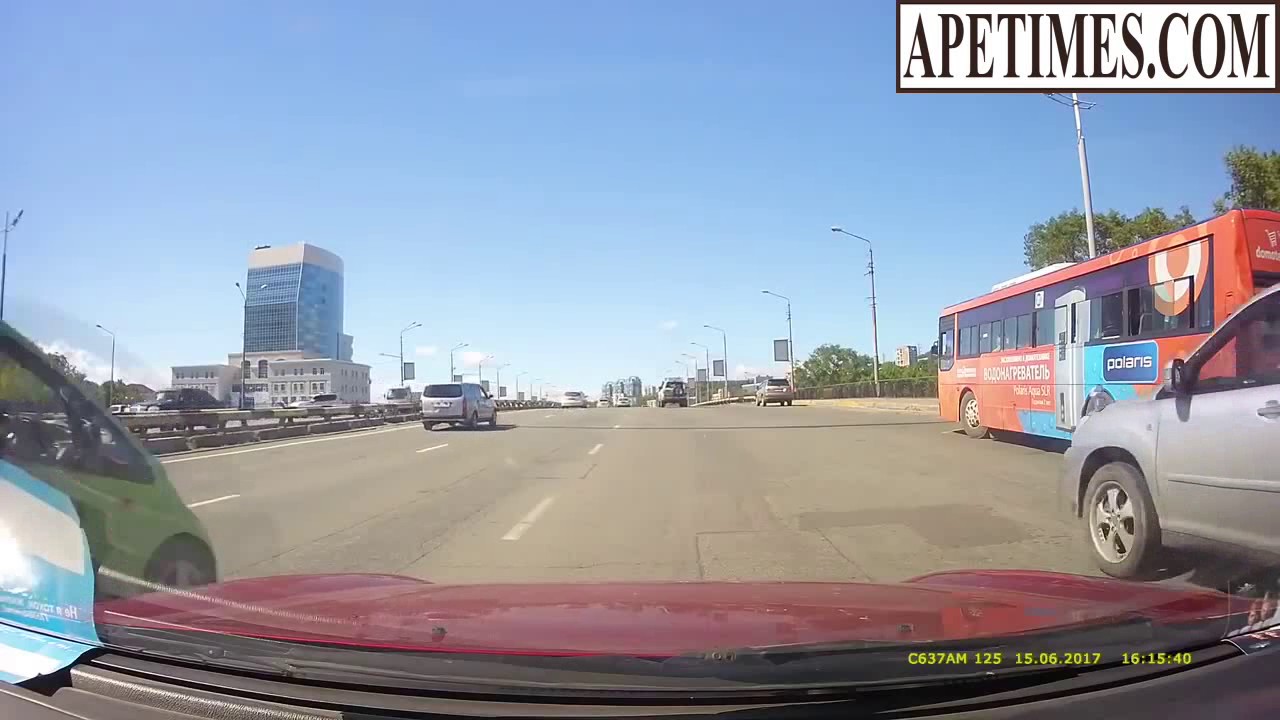This horizontal, rectangular advertisement is captured from inside a red car, likely from a dashcam situated on the front passenger side seat. Prominently, in the upper right corner of the photo, there is a horizontal, white rectangular background with a black border and all-capital black font text that reads: "APE TIMES.COM." The scene ahead shows a multi-lane road, probably three to five lanes wide, with clearly visible lane-divider white dashed lines. A notable element in the image is the timestamp located in the lower right corner in yellow font: "C637AM 125 15.06.2017 16:15:40."

The red hood of the car is visible from the perspective, and numerous vehicles occupy the road. To the immediate right, there is a whitish-gray car, visible from halfway through the driver's door forward. Further right, an orange bus with white fonts is entirely visible. On the left side, you can see the front of a green car. More vehicles, including a gray minivan or SUV, are observed ahead on the road.

The street is lined on both sides by tall metal poles with streetlights. To the left, beyond a guardrail separating traffic directions, stands a tall building with blue-glass windows. Trees with green foliage extend over the orange bus, adding natural contrast to the urban scene. The atmosphere suggests the photo was taken during the daytime, highlighting the busy city traffic.